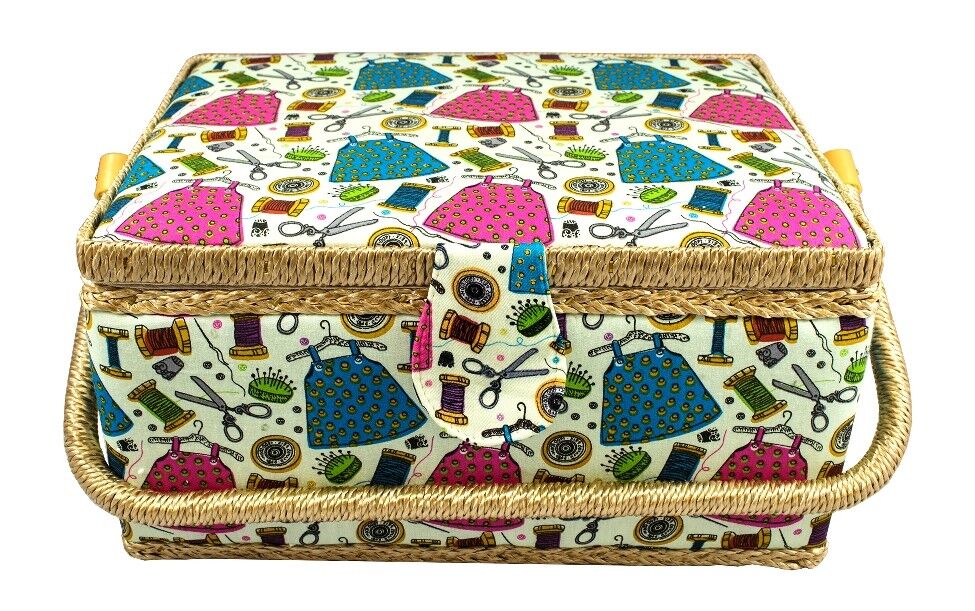This image features a square, woven sewing box with a handle, constructed from a combination of cloth and rattan materials. The box showcases a decorative cream fabric adorned with illustrations of sewing items including thread spools, scissors, needles, pin cushions, buttons, and hangers. The fabric spans across the top and front of the box, extending also to a Velcro fastening tab used to secure the lid. The edges of the box are lined with rattan trim, matching the material of the handle laid across its front. The rattan trim also accents the bottom of the box. Measuring approximately 12 inches wide and 4 to 5 inches tall, this meticulously detailed sewing box serves as a practical storage solution for sewing tools and materials.